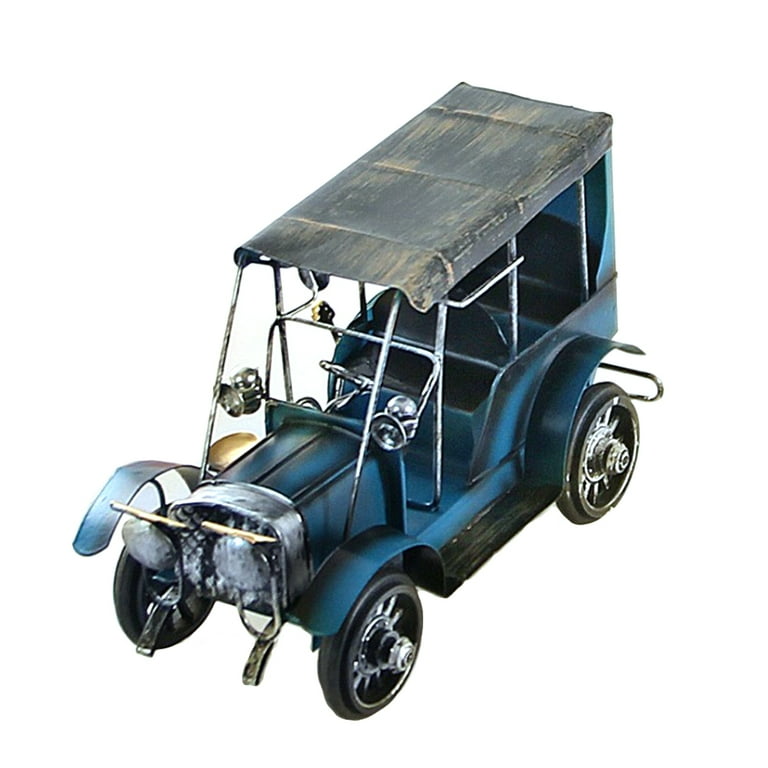The image captures a detailed model of a vintage vehicle resembling a Model T, viewed from a high angle close to 75 degrees, with its front facing the bottom left corner. The vehicle is set against a white background and boasts a light blue metallic body with a weathered, brown-copper canopy supported by metallic poles. The model exudes an immaculate level of craftsmanship with precision detailing, highlighting the chrome and gold components, including a small chrome steering wheel inside.

This vintage buggy, evocative of early 20th-century automobiles, features four black rubber-like tires with silver rims. The visible three of the four wheels, front headlights, a running board on the left side (our right), and dual side lights near where the windshield frame would be add to its authenticity. However, it is notably open, lacking doors, consistent with early car designs. The interior showcases two black bench seats, front and back, amid fine detailing with elements like a horn, grill, bumpers, and neatly crafted chrome pieces. The canopy, which could be perceived as a fabric or metallic tarp, complements its antiquated charm, underscoring the high craftsmanship of this exquisite model.